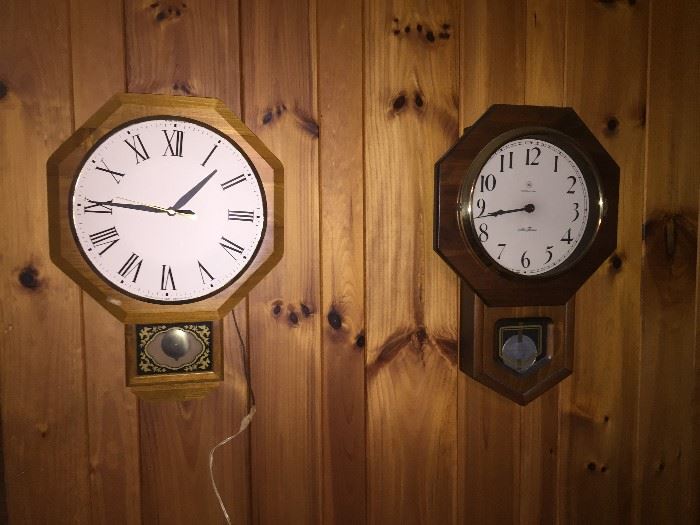The image is horizontally oriented and features two wooden wall clocks mounted side by side on a pine panel wall. The clock on the left is an electrically operated model with an octagonal bezel frame. The clock face is white and adorned with black Roman numerals, accompanied by a black hour and minute hand, and a gold-colored second hand. The small rectangular area below houses the pendulum. The time displayed is 1:46.

Adjacent to it on the right is a darker brown, battery-operated clock with a modern aesthetic. The octagonal frame of this clock has a gold bezel encircling the white clock face, which features contemporary numbers from 1 to 12. The black hour and minute hands show the time as 8:43. This Seth Thomas clock also includes a long, rectangular-shaped base extending down to a pointed end to accommodate the pendulum.